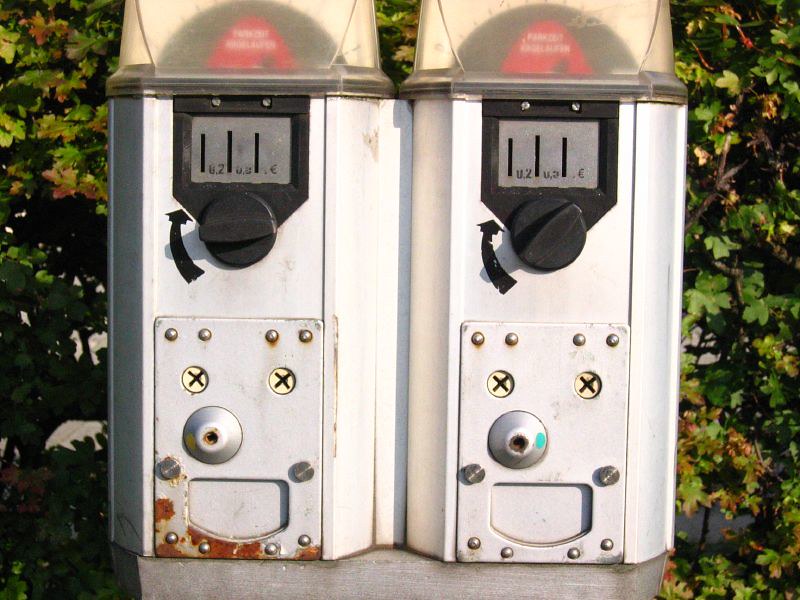In this photograph, we see two side-by-side white parking meters, possibly electric or coin-operated meters, that bear the appearance of faces. Both meters sit atop a metal pole and feature distinct facial-like details: the "eyes" are two circles with X-shaped pupils, a central knob resembles a nose, bolts on the left and right sides suggest cheeks, and a wide rectangular opening at the bottom forms a mouth, with additional bolts positioned like a chin. The parking meter on the left is rusted, whereas the one on the right appears cleaner. 

The meters also include various functional features. At the top, we observe a black dial with an arrow pointing upwards, along with three coin slots positioned below. A small plastic cover likely protects the meter reading. The base of each meter is a light gray color, transitioning to a slightly lighter silver-white hue above. Additionally, there's a trapezoidal door likely designed to dispense objects or change.

In the background, we see green leaves with slight browning, suggesting a natural setting such as a park or a leafy street. The overall scene provides a slightly whimsical yet functional urban snapshot, set against a verdant backdrop.